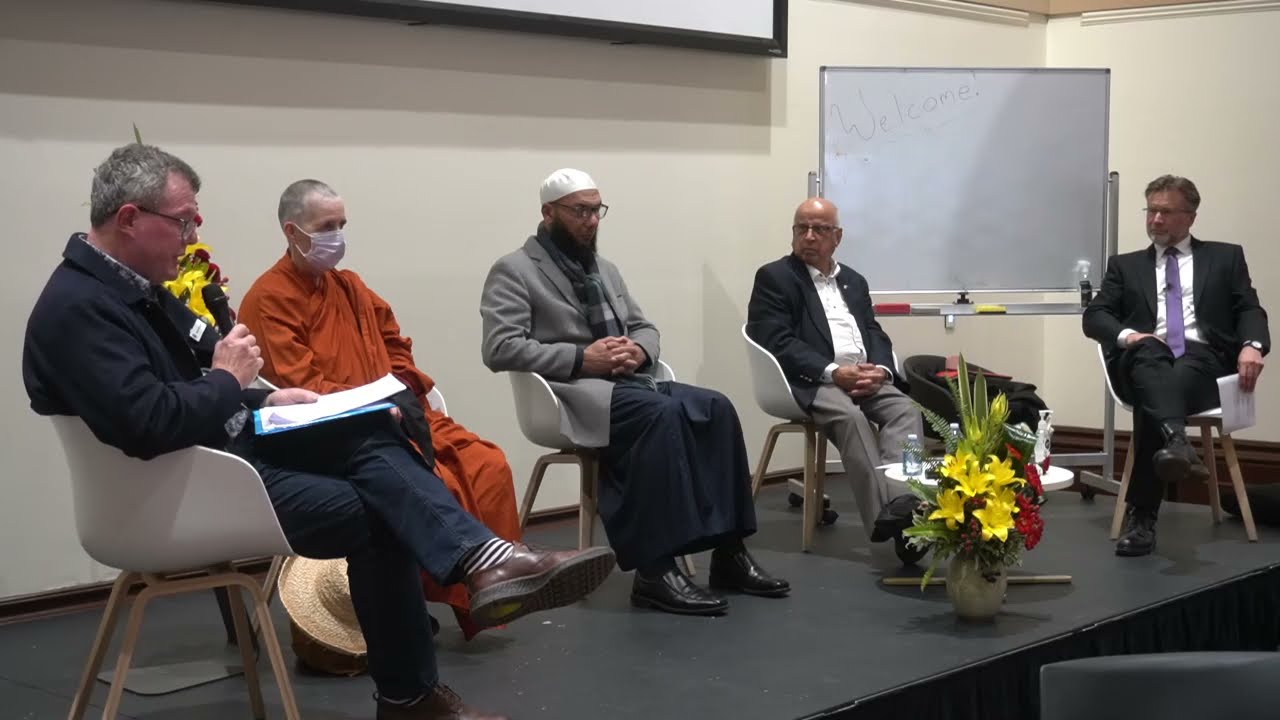This detailed color photograph captures an interfaith panel discussion on a dark charcoal grey stage, where five men of varying religious backgrounds are seated in a semi-circle on white plastic chairs. The stage backdrop consists of a tan wall, with a whiteboard in the right corner bearing the word "welcome" in its upper left corner. Behind the men, there is a blackboard between two white walls, and the top edge of what appears to be a projector or screen.

Starting from the left, the first man is dressed in a traditional suit with striped blue and white socks, brown leather shoes, and glasses. He is holding a microphone in one hand and reading from a white paper with his legs crossed, presenting something to an unseen audience. 

Next to him, the second man wears a vibrant orange robe, suggestive of a Buddhist monk, and a white face mask. His head is mostly shaved, and he listens attentively.

The third individual, positioned in the center, appears to be an imam. He wears a white skull cap, glasses, a gray suit jacket, and a traditional black dress-like garment. His hands are interlocked on his lap, signaling a contemplative and respectful presence.

To his right, the fourth man has a darker complexion, with a bald head and a bit of white hair. He is casually dressed in a white shirt and black suit jacket, sitting with his legs stretched out and hands clasped in front of him.

The fifth and final man, seated at the far right, sports a full head of black hair, dark glasses, a mustache, and a beard with gray streaks. He is formally dressed in a black suit, a white dress shirt, a long purple tie, and a fancy watch. His legs are crossed, and he focuses his attention on the man with the microphone.

Adding to the scene's color and atmosphere are two flower arrangements: one between the first and second men, and another between the fourth and fifth men. These arrangements consist of lilies and other red and yellow flowers, possibly indicating a summer or fall event. The setting and attire of the participants suggest a community meeting or conference among religious leaders, fostering dialogue and cooperation among different faiths.